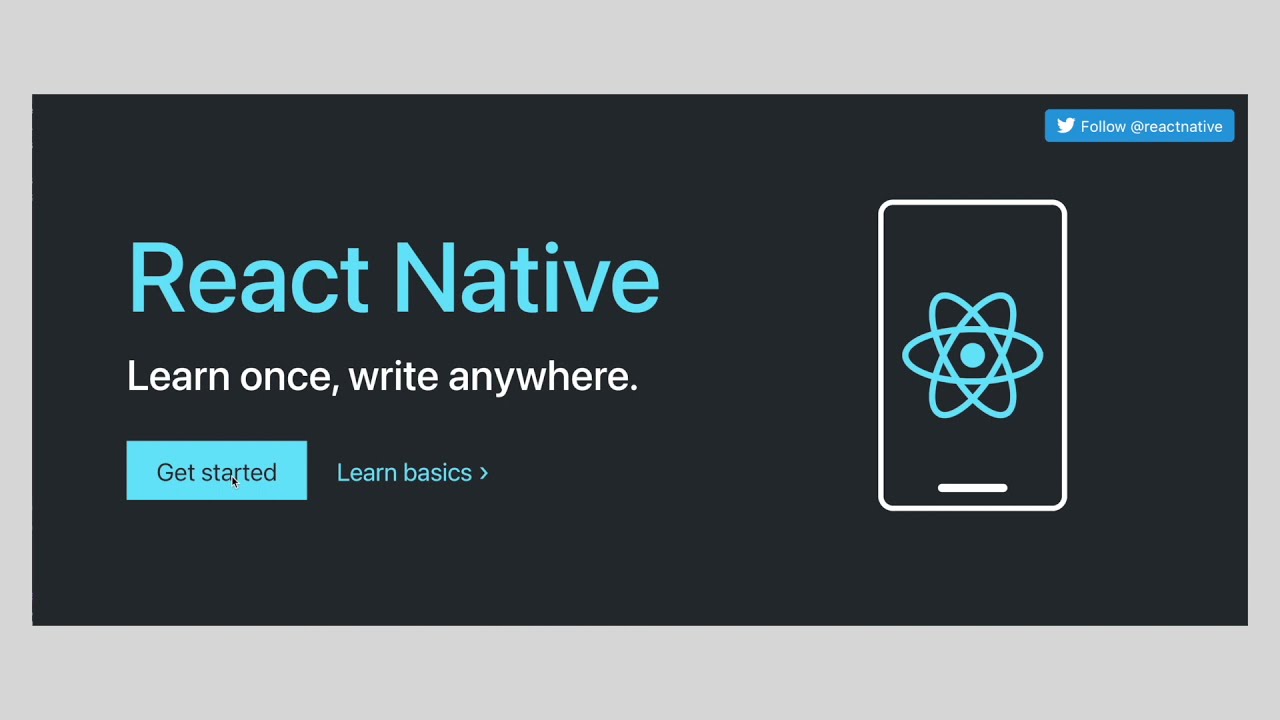The image depicts a sleek, black-themed webpage prominently displaying the text "React Native" in a large, teal font on the right side. Below this headline, a white subheading reads "Learn Once, Write Anywhere." This text is housed within a teal-colored box. Additionally, below this subheading, there is a "Get Started" button in black letters, and next to it, a link in teal letters that says "Learn Basics" accompanied by a rightward-pointing arrow. 

To the right, there is an image of a cell phone featuring a white outline. The phone screen displays a teal graphic of intersecting oval shapes. In the top-right corner of this image, the words "React Native" are shown alongside an icon similar to the Twitter logo. The entire section is contained within a black box outlined by very light gray borders. The top and bottom borders of this box are thicker, while the side borders are thinner. The overall design is clean, easy to read, and easy to follow.